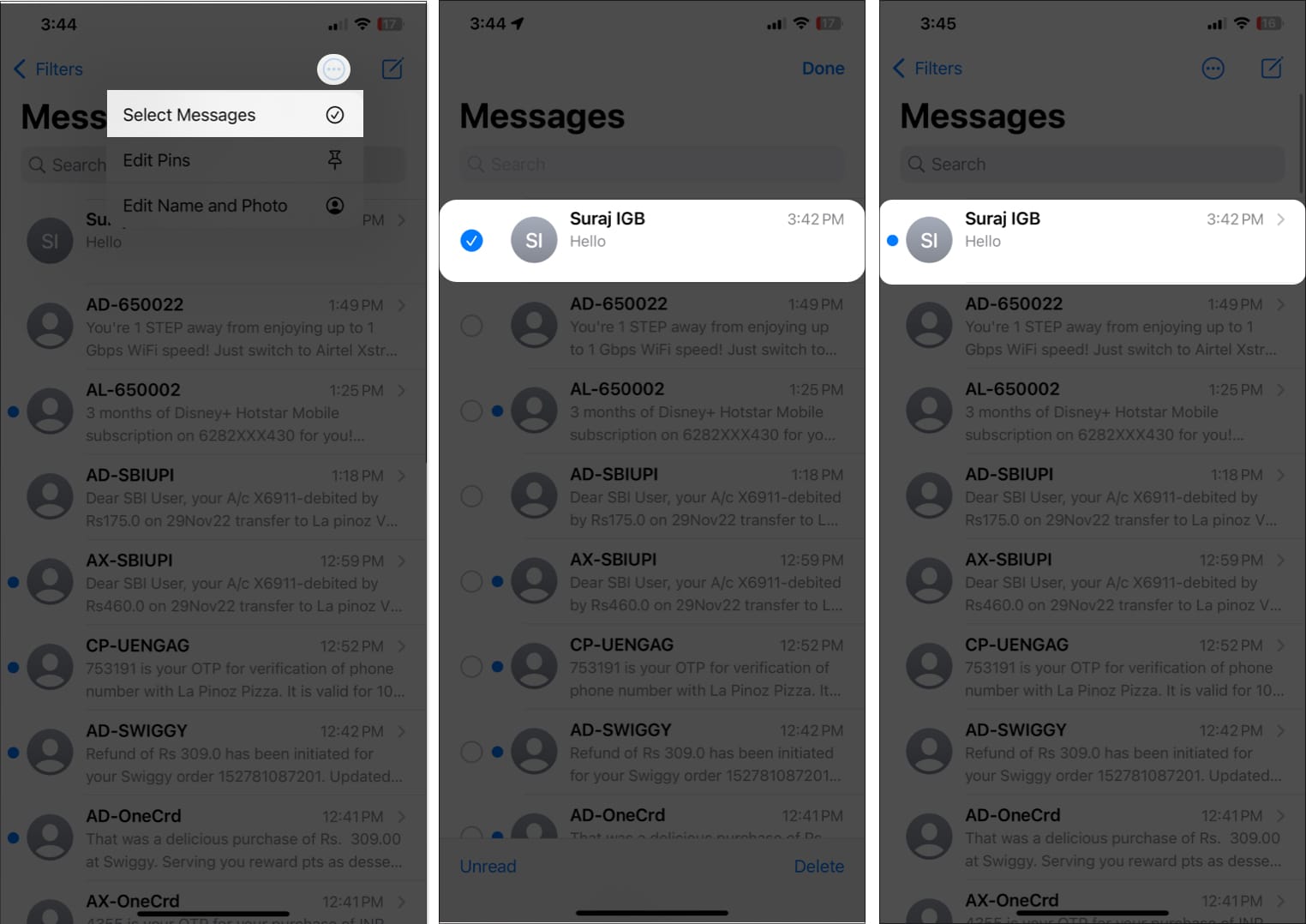### Detailed Caption for the Image:

The image displays three sequential smartphone screenshots placed side by side, each timestamped and featuring various interface elements. Moving from left to right:

1. **Leftmost Screenshot:**
   - **Time:** 3:44 PM
   - **Battery Level:** 17%
   - **Filter:** A blue filter is active above the Messages app.
   - **Pop-up:** A notification pop-up appears, saying “Select messages” in black text.
   - **Content:** The background shows a message received at 1:49 PM from "AD-650022," stating: “You’re one step away from a joining up to 1 Gbps Wi-Fi speed, just switch to RTL-XSTR ...”

2. **Middle Screenshot:**
   - **Time:** 3:44 PM
   - **Battery Level:** 17%
   - **Filter:** No blue filter is present.
   - **Pop-up:** The pop-up displays a message from "Siraj, IGB" sent at 3:42 PM, which reads “Hello.”
   - **Content:** Similar to the first screenshot but without any highlighted filters.

3. **Rightmost Screenshot:**
   - **Time:** 3:45 PM
   - **Battery Level:** 16%
   - **Filter:** A blue filter is again present above the Messages app.
   - **Pop-up:** This shows the same message as in the middle screenshot from "Siraj, IGB,” also sent at 3:42 PM.
   - **Content:** Additionally, shows a message received at 1:25 PM offering a “three months of Disney Plus Hotstar mobile subscription...” followed by a series of numbers and letters: "16282XXXX4304U."

All three screenshots share a consistent dark gray backdrop caused by the appearance of the notification pop-up. Blocks of black and gray text can be observed, predominately containing timestamped messages from various sources, including promotional and informational content featuring alphanumeric codes and URLs.